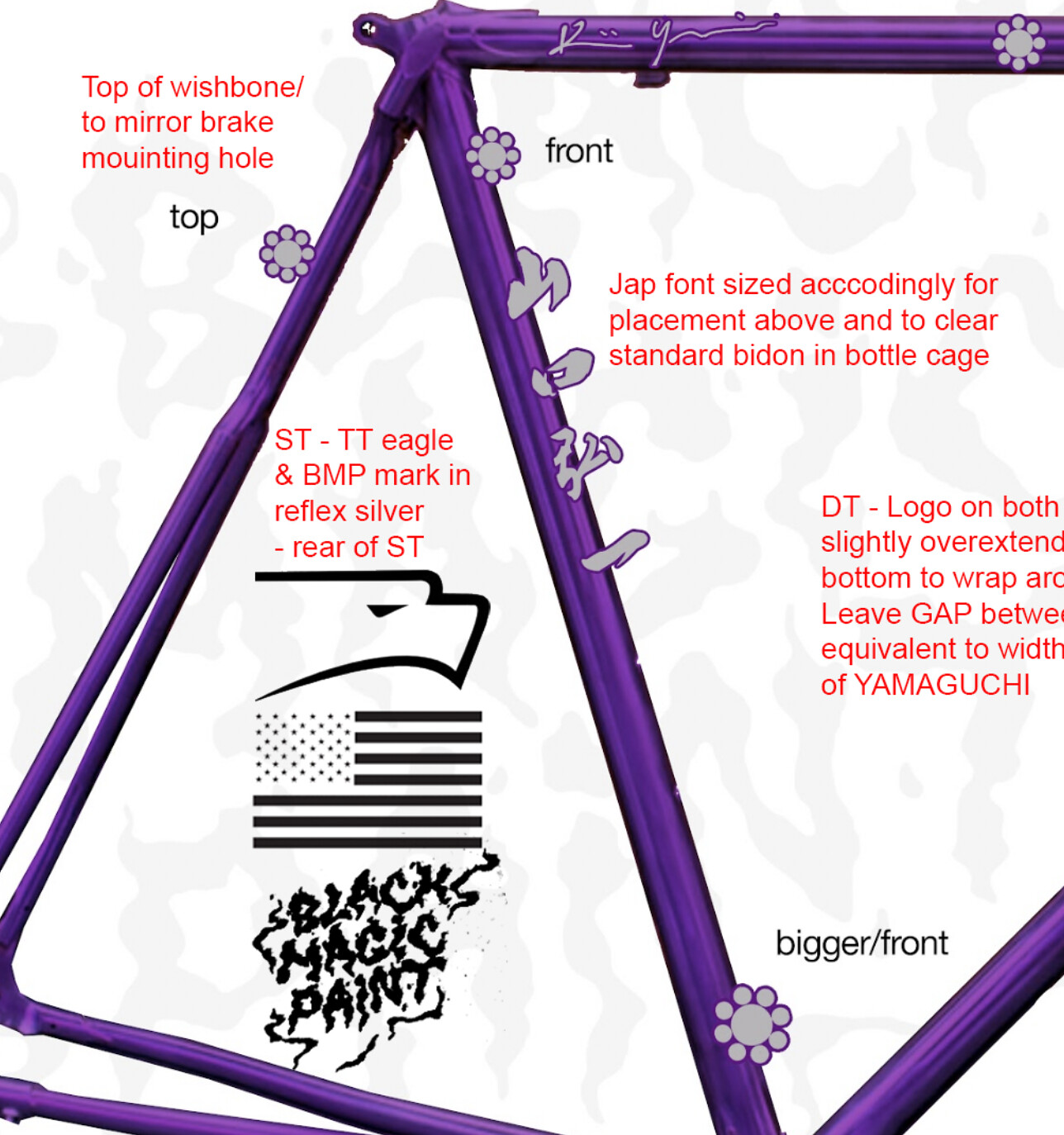The image appears to be an instructional pamphlet showing how to assemble or place various elements, possibly related to a park or a device. Central in the image is an American flag with an eagle above it. The background showcases a gradient of colors including white, tan, black, purple, gray, and red. The text is spread all over the image and is not centered, contributing to a somewhat chaotic layout. Prominent phrases in both red and black text include: "top of wishbone to mirror brake mounting hole," "ST, TT Eagle, and BMP marked in reflex silver, rear of ST," and "DT logo on both, slightly overextended bottom to wrap and leave gap equivalent to width of Yamaguchi." Additional instructions mention font placement for a "jab front" and accommodating a standard bidon and bottle cage. The presence of purple stripes forming a triangle, along with silver and flower symbols, adds to the detailed yet cluttered design.